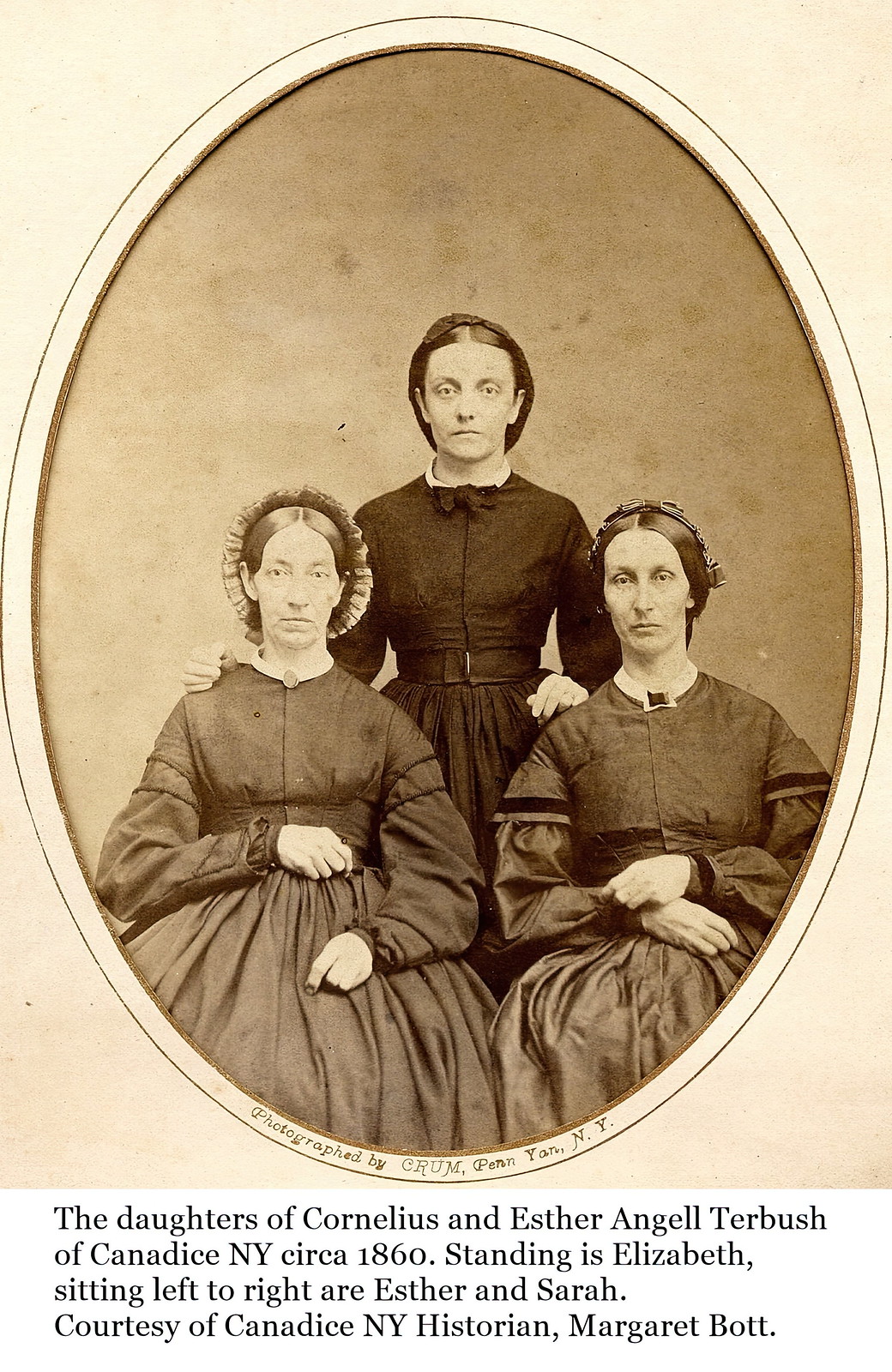The image is a sepia-toned photograph from circa 1860, displayed in an oval white frame with black cursive writing that identifies the photographer as Crum, Penn, New York, NY. The photo captures three women dressed in Victorian-era outfits, indicative of the 1860s, with their stern faces and hair pulled back, adorned with braids or bonnets. The central figure, standing, is Elizabeth, wearing a dark outfit. Sitting on either side of her, with their hands crossed in front, are Esther (left) and Sarah (right). Beneath the photograph, a caption in black font reads: "The daughters of Cornelius and Esther Angell Turbrush of Candace, NY, circa 1860. Standing is Elizabeth. Sitting left to right are Esther and Sarah, courtesy of Candace, NY, historian Margaret Bott." The overall photograph rests on a beige background, further accentuating its antique quality.